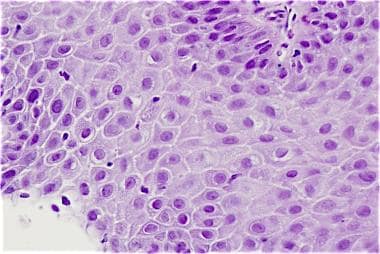This highly magnified color photograph, possibly viewed through a microscope, depicts a densely packed array of rounded, cell-like structures varying in shades of purple. The image features thousands of these cells, each distinctly visible with their own light purple centers encircled by a thin white border, and darker purple nuclei. The cells are set against a predominantly white background, with a notable clear and lighter purple center, while the left side near the bottom shows darker purple hues. In the lower left, there is a small section of white space, and the top right corner displays a cluster of purple circles bordered by clear fills and enveloped in white lines, also showing a slight wrinkle descending from the upper right. The overall composition is intricate, with significant detail highlighting the variation in color and structure within the cells, which could either suggest a microscopic slide or an abstract artistic representation.